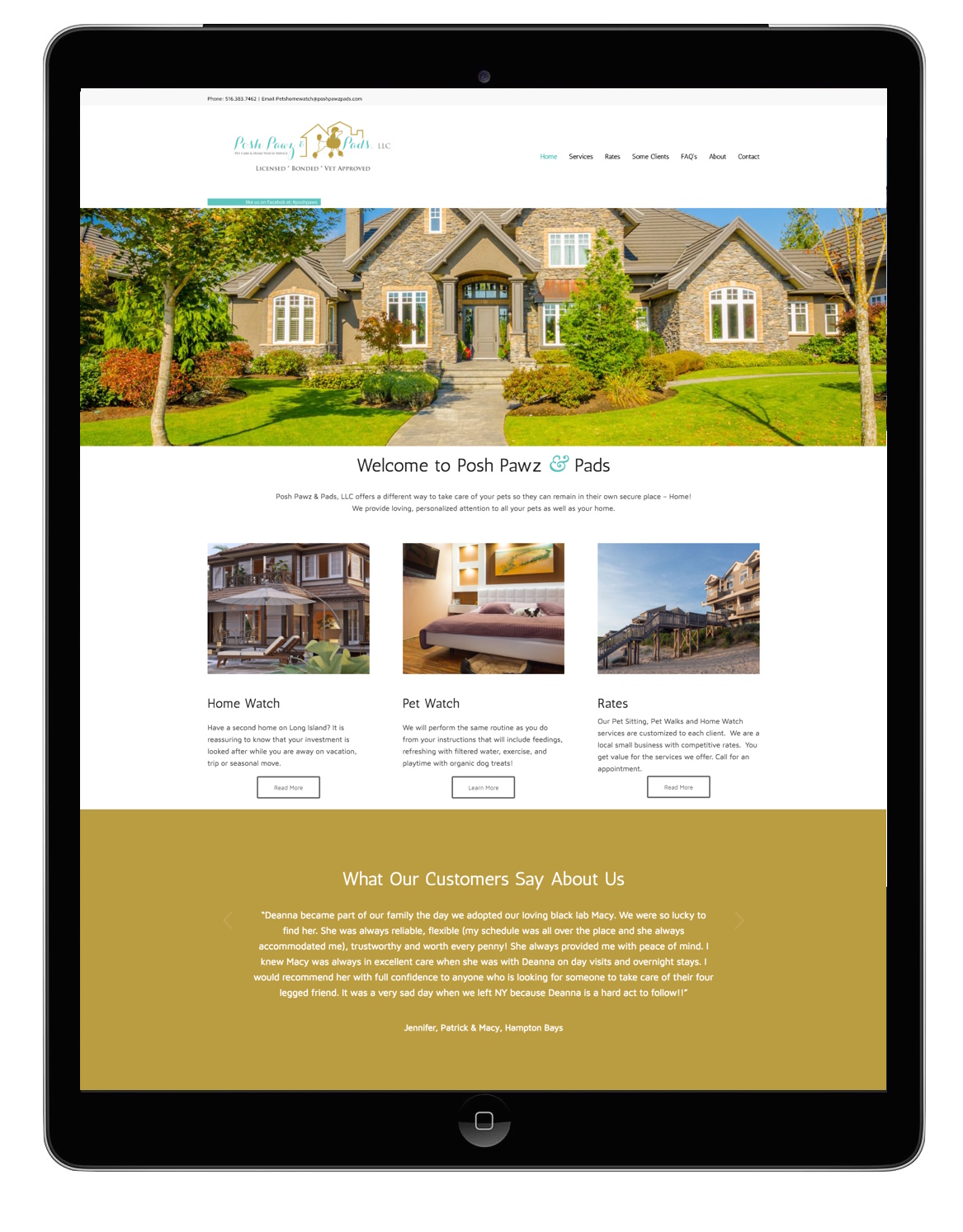The screenshot depicts a section of a mobile app for "Posh Paws and Pads." The app features a stylish header with a light teal cursive logo that reads "Posh Paws and Pads," accompanied by an outline of a house with a poodle in front of it. The primary image shows an opulent home with a beautifully manicured and landscaped yard, including neatly trimmed trees and a wide sidewalk leading to the entrance. This suggests that the service caters to high-end real estate.

The app offers three main options: Home Watch, Pet Watch, and Rates, implying services for overseeing homes and pets. These features suggest that Posh Paws and Pads provides caretaking services for homeowners and pet owners, particularly those who own luxurious properties. Below these options, there's a testimonial section where a customer's feedback starts with, "What do our customers say about it?" One testimonial visible reads, "One of their workers became part of our family the day we adopted our...", hinting at the personalized and familial nature of the provided services. Overall, the app appears to target affluent individuals looking for premium home and pet care.